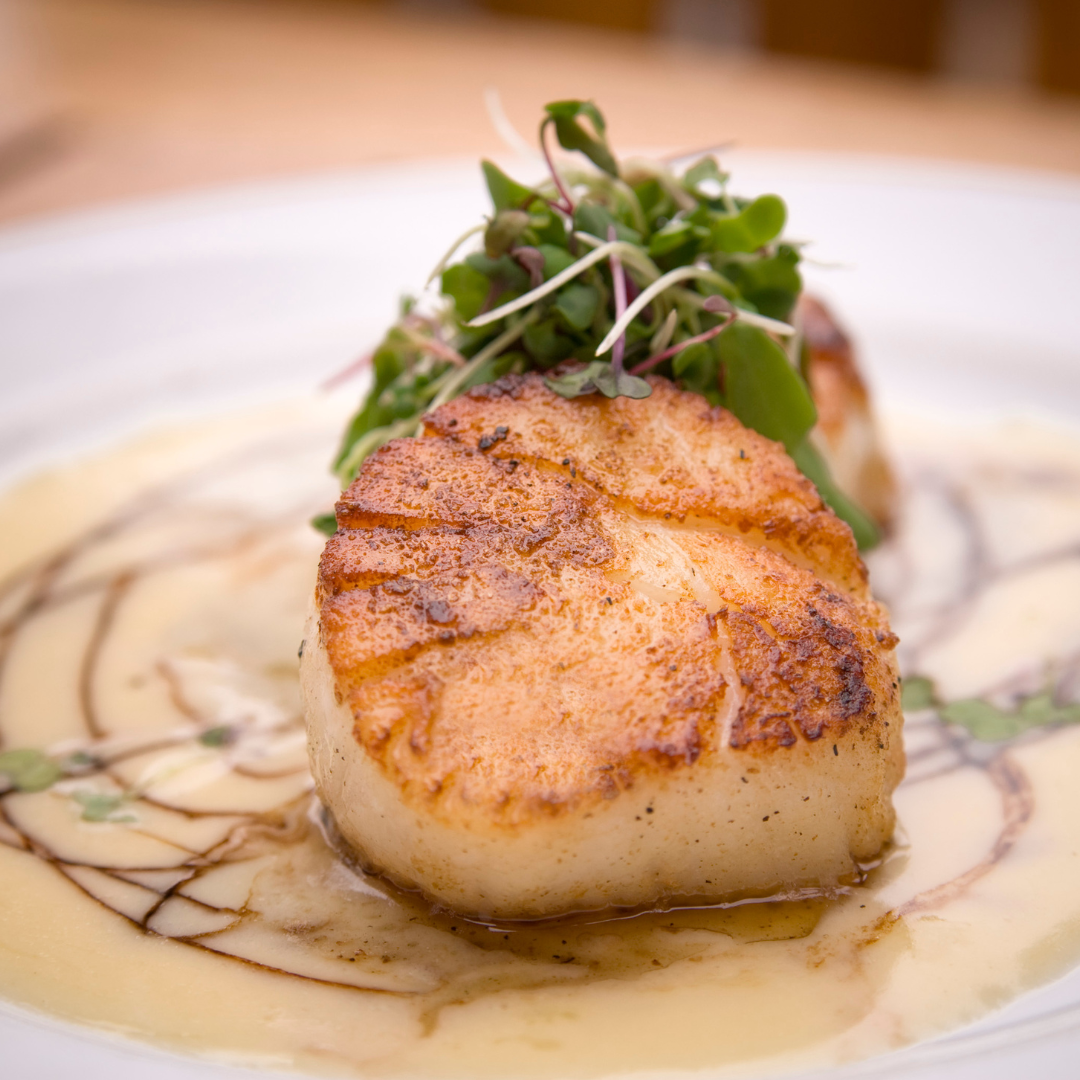The image showcases a gourmet dish that appears to have been photographed in a fine dining setting. The central focus of the dish is a piece of lightly browned and grilled white fish or possibly a scallop, with a golden-orange tint and slight caramelization on top. The protein rests on a light-colored, pancake-like base, which has a glossy sheen indicative of some syrup or sauce. Adding to the visual appeal, the dish includes a garnish of green leaves, potentially parsley or sprigs of lettuce, along with vivid accents of white and pink, likely sprouting greens. The white plate serving the food is adorned with an artistic arrangement of cream or fish sauce, featuring intricate circular patterns of brown and green streaks, showcasing deliberate and creative presentation. The background is slightly blurred, including a glimpse of a brown table edge and a darker brown wall, enhancing the focus on the meticulously arranged dish.